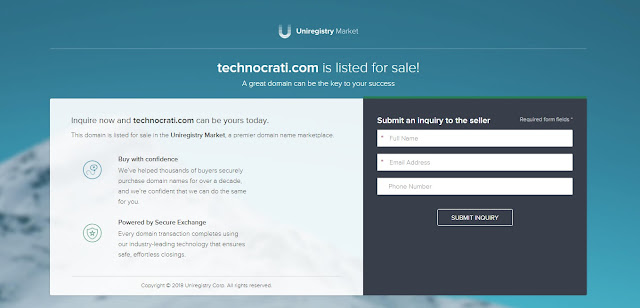The image is a screenshot of a web page, prominently conveying that a domain name, technocrat e.com, is available for sale. The entire background features a gradient from a dark blue to a lighter blue, with what seems to be a blurred close-up image of a mountain peak set against the dark blue sky.

At the top center of the page, there is a logo consisting of a "U" icon, followed by the text "Uniregistry." Beneath the logo, a thin white line separates the header from the main content. In bold letters, "Technocrat e.com" is displayed at the center, immediately followed by the phrase "is listed for sale!" Below this, a subtext in smaller font reads, "A great domain can be the key to your success."

The page is divided into two main sections: the left section is a slightly transparent white box, while the right section is a dark blue, nearly black box.

In the left section, the text reads, "Inquire now" and "technocrat e.com can be yours today." There is smaller, unreadable text beneath this. Further down, two subsections are labeled. The first subsection, titled "Buy with confidence," comes with an icon to its left and four lines of text. The second subsection, labeled "Powered by secure exchange," also features an icon to its left, accompanied by three lines of text. At the very bottom of this section, a line separates the content, and below this, it states, "© 2004 Uniregistry.com," in very small text.

In the right section, within the dark box, there is a form titled "Submit an inquiry to the seller." The form is comprised of three fields asking for your full name, email address, and phone number. Beneath these fields, there is a "Submit Inquiry" button.